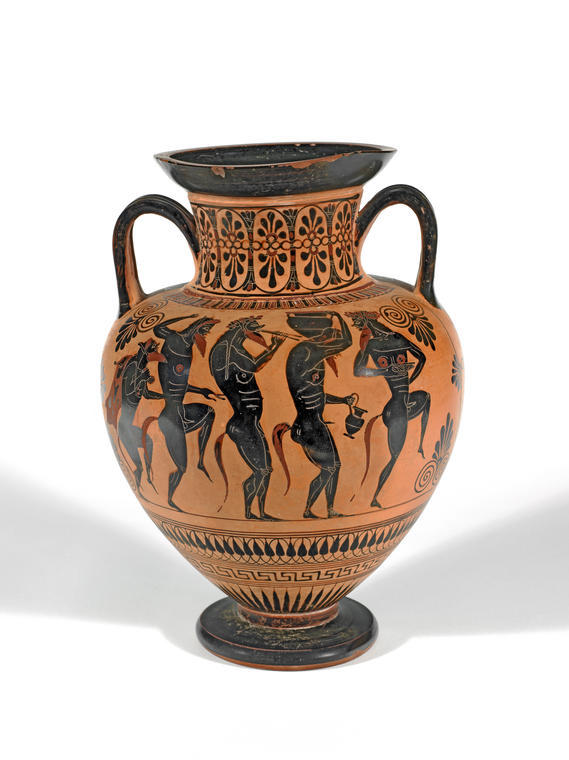The image depicts an ancient Grecian urn, seemingly made of terracotta, featuring a tan base color with intricate black designs. The urn has a wide, bulging body that tapers towards a black foot, with dual black handles attached at the neck's sides. The mouth is distinctively black, transitioning into a short, wide neck decorated with black and red circular patterns. Prominent in the urn's design are five bearded centaurs, each participating in a dynamic procession from left to right, which is characteristic of traditional Grecian artwork. The centaurs are depicted with dark skin and orange beards and tails. The leader points to the right but looks back at his companions, adding a sense of narrative to their movement. The second centaur carries a vase on his head; the third plays a wind instrument; the fourth holds a basket in one hand and a bowl in the other; while the last centaur, adorned with a wreath, is distinguished by slightly reddish chests and also looks back. The urn rests against a white background with a shadow cast diagonally from the bottom left to the bottom right, emphasizing its three-dimensional form. This urn exemplifies the ornate and functional artistry of its time, likely used for transporting water or other liquids.